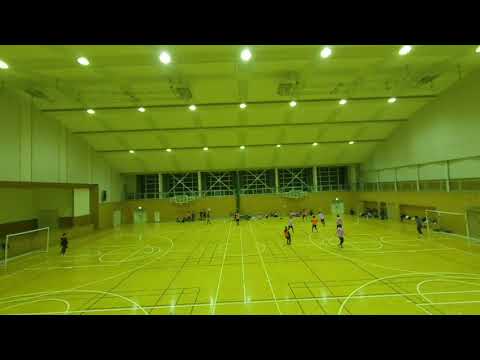The image depicts the interior of a school gymnasium at night, with its yellowish-orange floor prominently marked with various intersecting lines for multiple sports, indicating a multi-purpose use including basketball, floor hockey, and soccer. On either side of the gym, soccer goals are set up, with a few children engaged in a game, although no ball is visible. The gymnasium is illuminated by rows of overhead lights, and its walls are light white, transitioning to an orange-yellow hue at the bottom. The high, light-colored ceiling also features these lights. The far end of the gym is lined with black windows, suggesting it is night outside, and students can be seen sitting on a brick wall beneath these windows. Additionally, basketball hoops are faintly visible in the background, underscoring the gymnasium's versatility. There are several doors along the walls, indicating access to other areas, and an opening on the left that likely leads to a hallway or entrance.